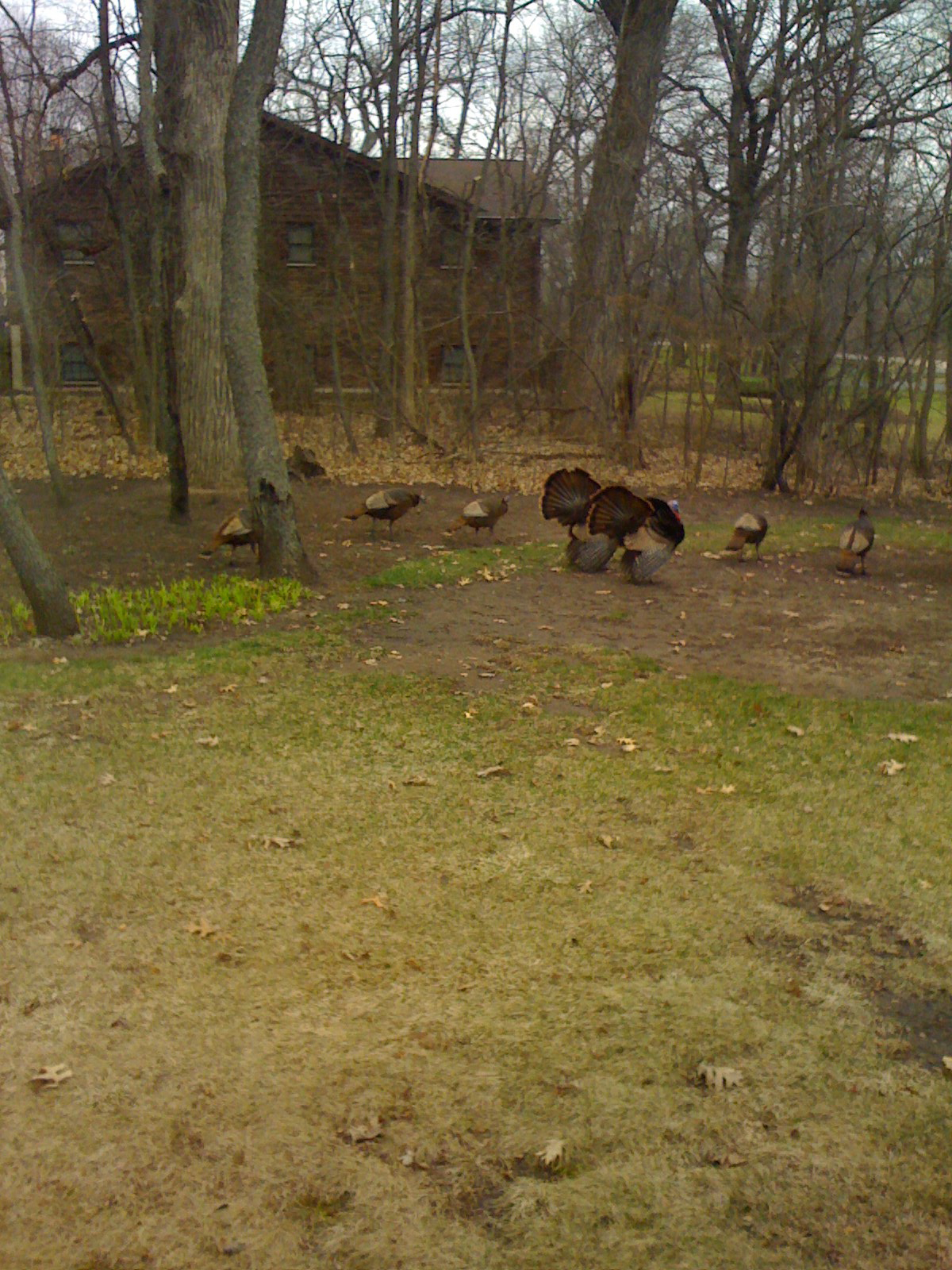The daytime outdoor color photograph features a large two-story house with dark brown brick siding and a brown roof, situated in the background. The lawn in the foreground consists mostly of patches of dull light green grass, interspersed with dirt areas and scattered brown and yellow leaves, evidencing the seasonal transition. Prominent towards the center and slightly right of middle, the scene captures about eight to nine wild turkeys, most notably two with their wings raised, exhibiting intricate patterns of dark brown and light brown feathers. Some turkeys pick at the ground while others strut across the dirt patch. The background is accentuated by tall trees, lending height and depth to the image, although the trees are barren of leaves, their branches stark against the overcast sky. The scene is imbued with a natural palette, creating a harmonious yet slightly blurred image that focuses on the rustic outdoor setting and the wildlife inhabiting it.